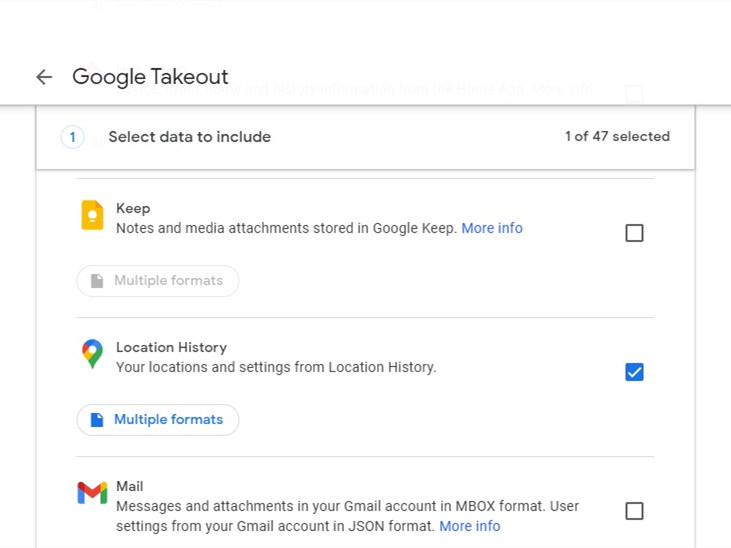This is a detailed screenshot of a Google Takeout interface, specifically the "Select data to include" section. Here, the user has opted to select only one of the available 47 data categories for export. 

The first highlighted selection is "Google Keep," indicated by a yellow box featuring a light bulb icon. This section includes notes and media attachments stored within Google Keep.

Directly below, there is another selection for "Location History," detailing the user's locations and settings from the "Location History" feature. Next to this, there is a white button with blue text that reads "Multiple formats," which is currently checked.

The next data category visible is "Mail," distinguished by an envelope icon. This category encompasses email messages and attachments from the user's Google account. Accompanying this, there is information about user settings in the Google account, designated to be exported in JSON format.

Additionally, there is a "More info" link in blue text, likely providing further details about the data being exported. This interface snapshot showcases the versatility and granularity of the data export options available via Google Takeout.